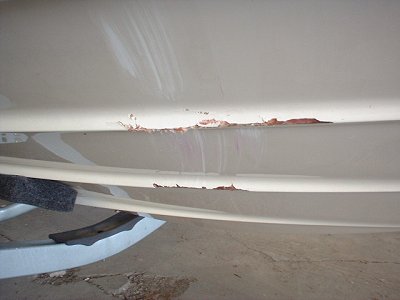In this detailed and closely-cropped image, the focus is on three horizontal beams that appear to be made of either metal or plastic, given their sheen and creamy beige color. These beams, which may be components of a larger structure such as a boat lift or scaffolding, show significant wear with visible brown exposed metal where the paint has been scraped away. They are situated above what looks like a concrete floor, which reinforces the industrial or repair setting of the image. To the left, there is a vertical, white bracing or structural support, while in the background a white-painted wall has additional streaks and smudges of white paint. Also present in the scene is a black object resembling a paint roller with a white handle, and another white piece with a black rectangular marking. The beams themselves look worn, possibly damaged, suggesting an environment concerned with maintenance or construction.